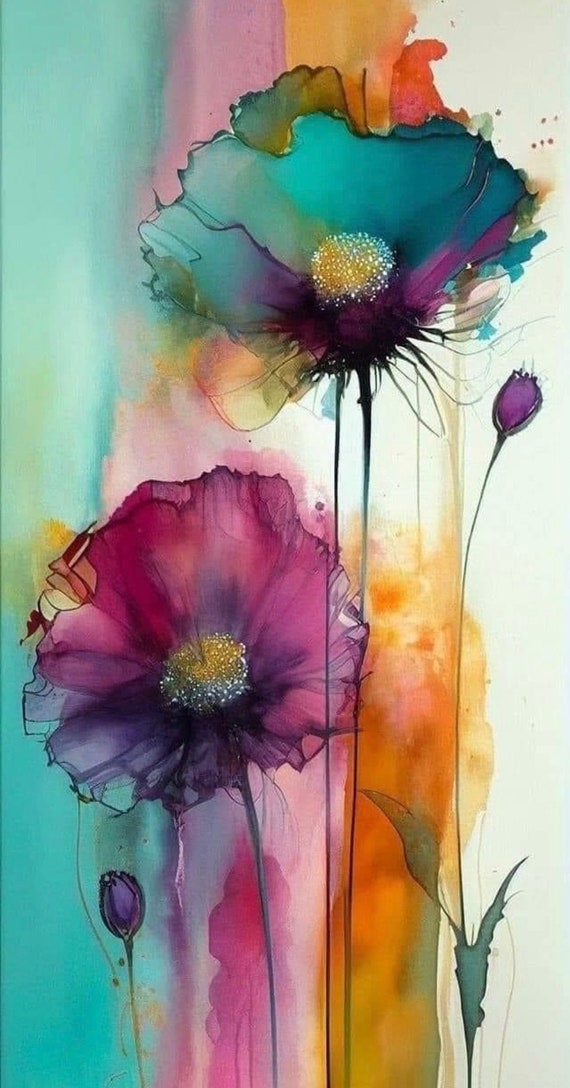This painting, a watercolor artwork, features an abstract depiction of flowers on a long, rectangular canvas positioned in portrait mode. At the center, two large flowers in full bloom dominate the scene. The flower on the left boasts fuchsia and purple petals with a mixed center of white and gold, making it shorter compared to the one on the right. The latter stands taller with petals in various shades of blue, some green tinges, and a yellow and white speckled center that appears glittery. Flanking these blooms are two smaller, unbloomed purple tulips—one situated to the left and the other to the right of the main flowers. The turndo right has visible green stems or leaves. The flowers' colors bleed beyond their petals, blending harmoniously to form a vibrant background filled with streaks of blue, purple, orange, and yellow. The right side of the painting remains mostly white, providing a stark contrast. Overall, this mass-produced, detailed watercolor composition incorporates a rich palette of aqua, gold, orange, pink, purple, and fuchsia, making it a vivid and dynamic abstract floral piece.